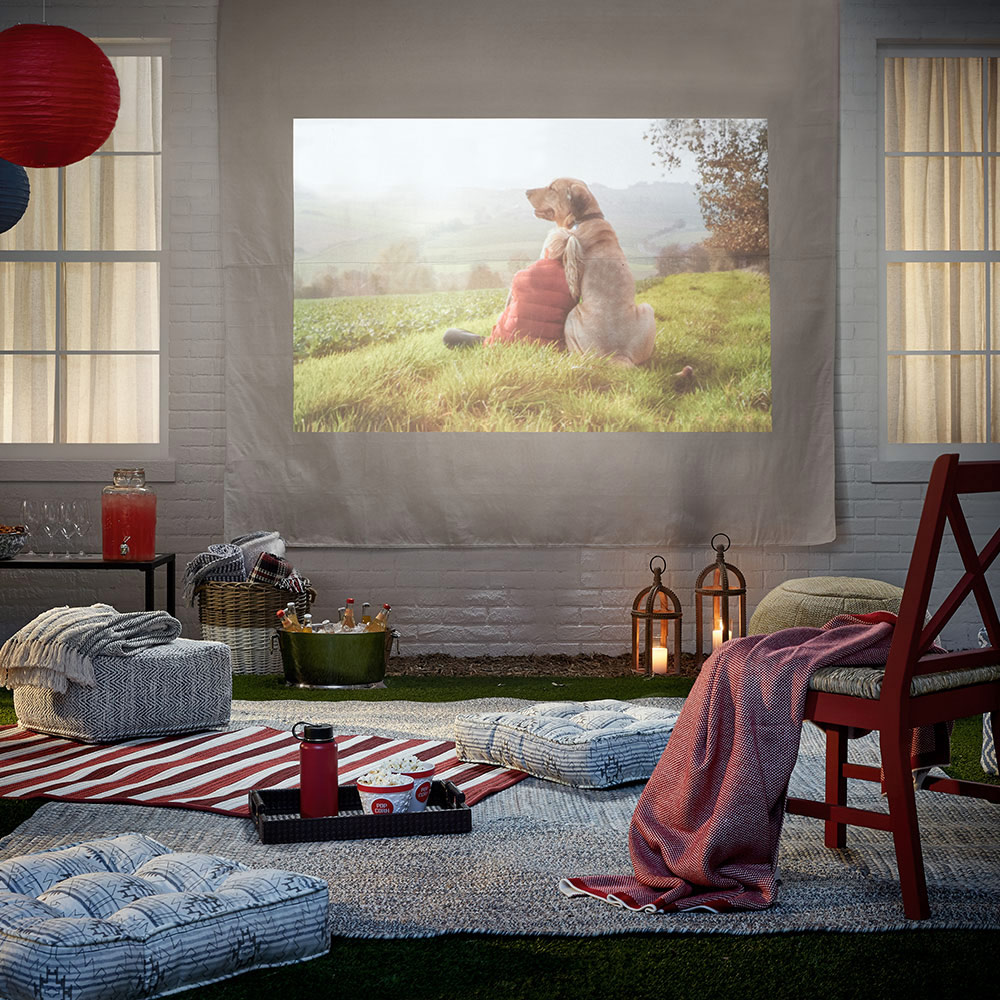The image vividly captures a cozy living room meticulously set up for a delightful slumber party. On the floor, a couple of cushions are arranged on top of a mat, providing a comfortable seating area. In front of the cushions, a black tray holds two cups brimming with popcorn, distinguished by their white and red rims. Additionally, a little red bottle with a black top, presumably containing a beverage, sits within the tray. Another rug features bold red and white stripes, adding to the lively ambiance.

A nearby red chair is thoughtfully adorned with a red blanket draped over its back, enhancing the room's warm color palette. Dominating the background is a projector screen displaying a serene movie scene of a blonde-haired woman in a red jacket cuddling a yellow Labrador Retriever in a grass meadow, immersing the room in a movie-watching atmosphere.

Further adding to the inviting setup, below the screen, there is an assortment of beverages accompanied by an ice bucket and a couple of candles, casting a soft, flickering glow that heightens the cozy ambiance.